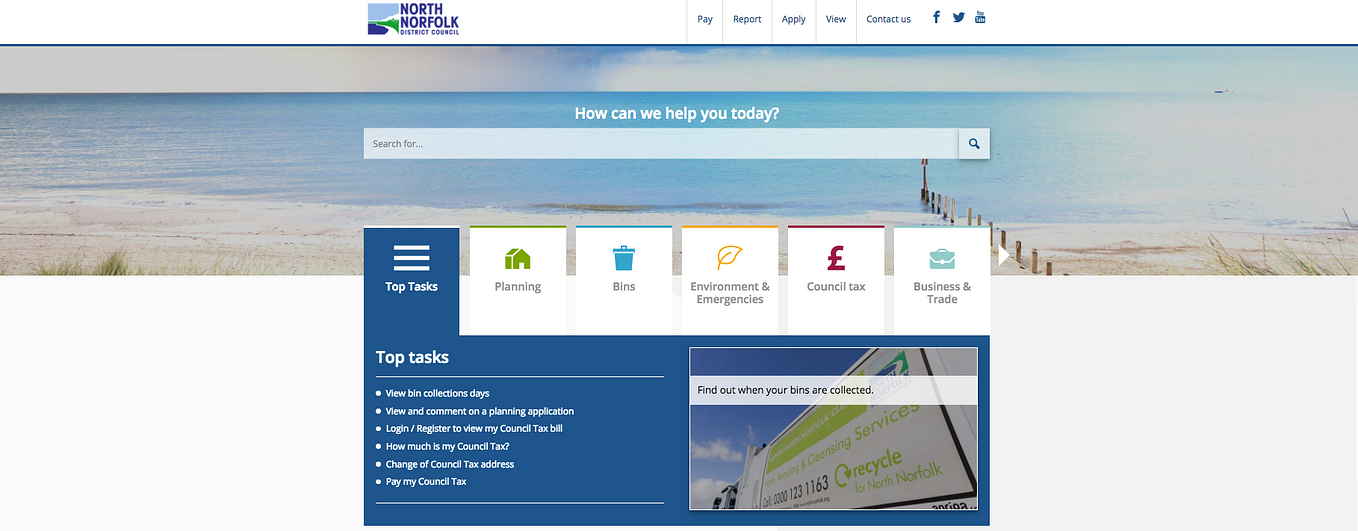This screenshot depicts the homepage of the North Norfolk District Council website. The header features a serene image of a beautiful beach, evoking a sense of the area's natural beauty. Directly below the header, a navigation bar offers quick access to essential functions with tabs labeled: "Pay," "Report," "Apply," "View," and "Contact Us." Additionally, icons for social media platforms such as Facebook, Twitter, and YouTube are prominently displayed at the top. 

Central to the page is a welcoming message, "How can we help you today?" positioned above a search bar inviting users to "Search for..." accompanied by a magnifying glass icon. Below this section, the website is organized to facilitate user needs with five clickable tabs: "Top Tasks," "Planning," "Bins, Environment and Emergencies," "Council Tax," and "Business and Trade."

The currently selected "Top Tasks" section lists seven frequently used services in bullet points:
- View bin collection days
- View and comment on a planning application
- Log in/register to view my council tax bill
- How much is my council tax?
- Change of council tax address
- Pay my council tax
- Find out when your bins are collected

The remaining content area has a clean white background, ensuring easy readability and navigation. This structured layout emphasizes the Council's commitment to providing accessible and efficient online services for its residents.